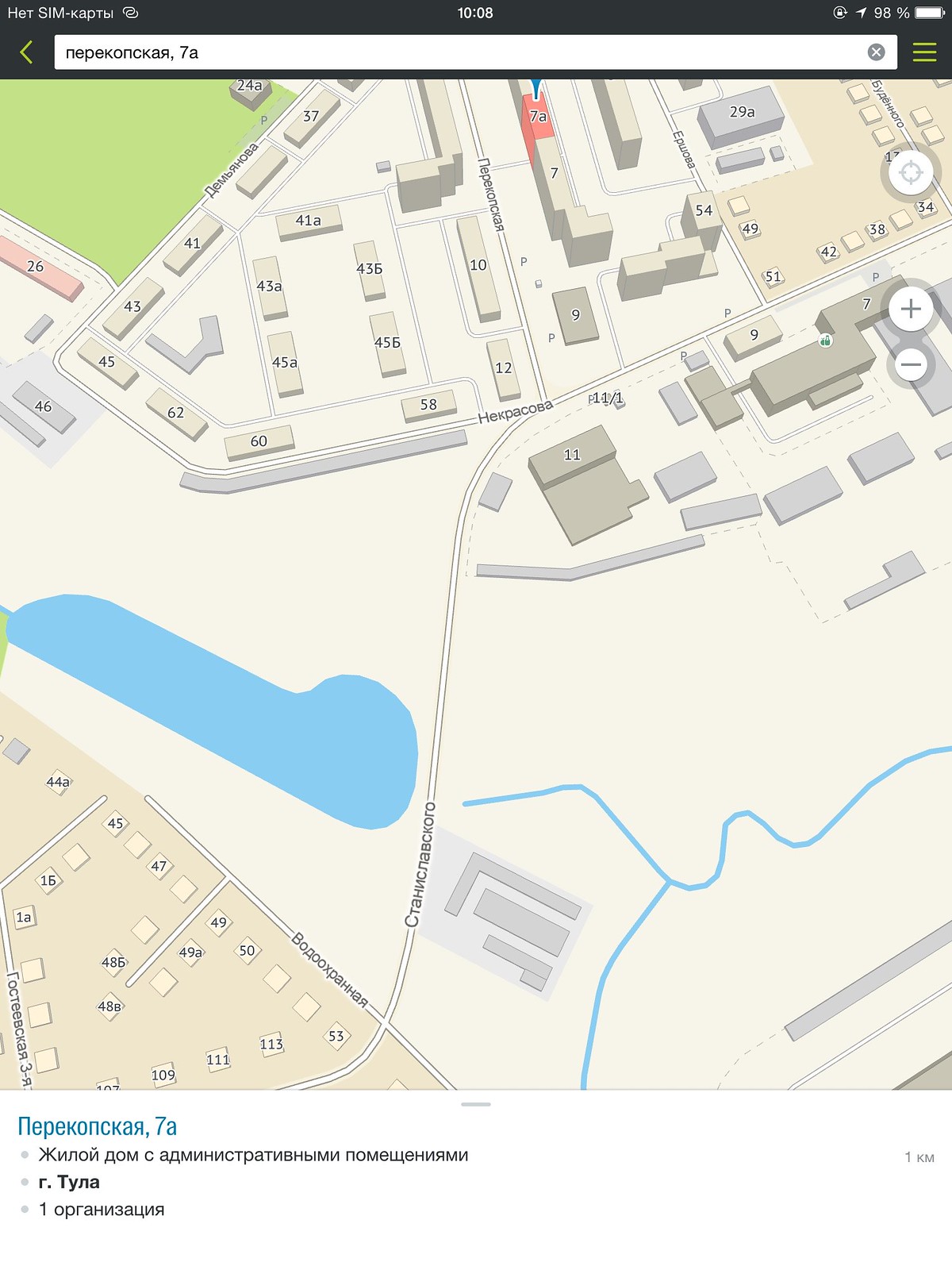This image is a screenshot taken from a phone, tablet, or computer. At the very top, there is a thin black bar stretching across the screen. In the upper left corner of the bar, white writing is visible, while the center displays the number "1008." The upper right corner of the bar contains several symbols, including a white rectangle representing a battery.

Below the black bar is a navigation bar. It features a left-pointing yellow arrow, followed by a thin white rectangular box containing Russian text. On the right side of this white box, there is a circle with an 'X' inside it. Adjacent to this, still within the gray background of the navigation bar but outside the white box, are three horizontal yellow lines.

Below the navigation bar lies a map. The map highlights a section of a city, showcasing various buildings, a significant body of water such as a lake or pond, and a small brook. Under the map is a white information bar with Russian writing, structured as a header followed by three bullet points.